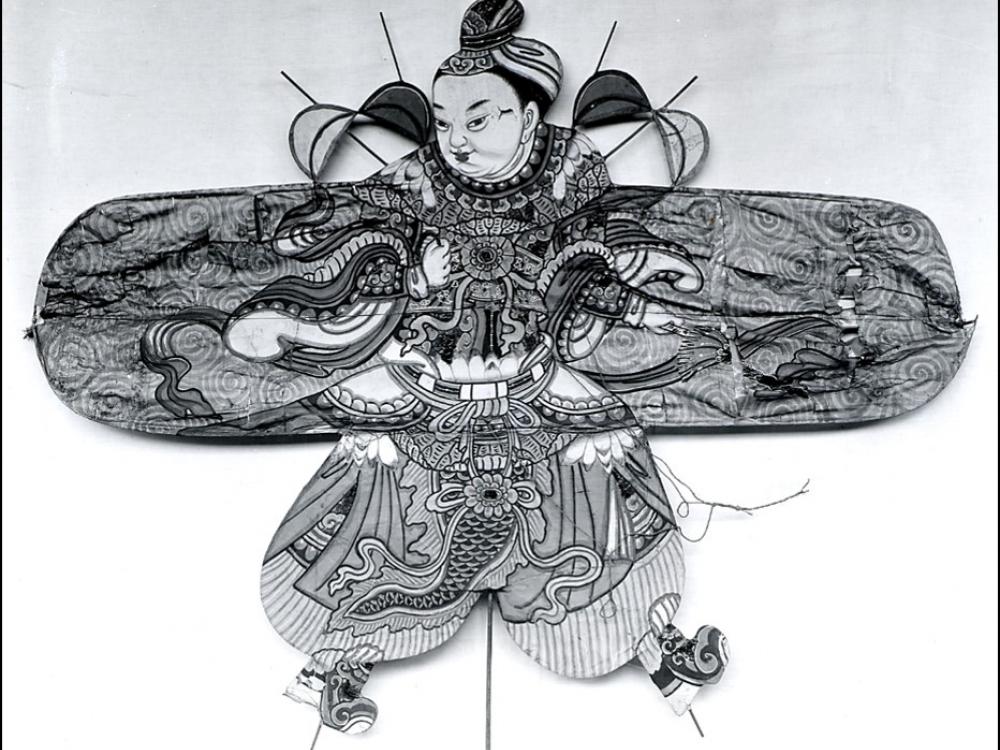In this black and white image, we see a detailed and ornate depiction of an Asian woman, likely an artistic piece from China. The woman, who has a round, chubby face with small lips and defined cheeks, is facing the seven o'clock position but looks directly at the viewer with her eyes. A high bun tied with a scarf adorns her head, and a jeweled band rests across her forehead. Her costume is highly intricate with fine details, featuring a combination of floral patterns, fish-scale-like textures, and squiggly lines resembling snakes. Her arms stretch out to the sides, connected to an oval-shaped torso, giving an exaggerated, caricature-like appearance. Her large, poofy pantaloons extend outward in a W shape towards delicately detailed boots. The entire costume, including hints of fingertips emerging from her sleeves, emphasizes the ornate and artistic craftsmanship involved, suggesting a rich layering of fabric and possibly paper. The woman's slight grin and the mixture of decorative elements showcase the elaborate, 3D design intended to captivate and draw attention.